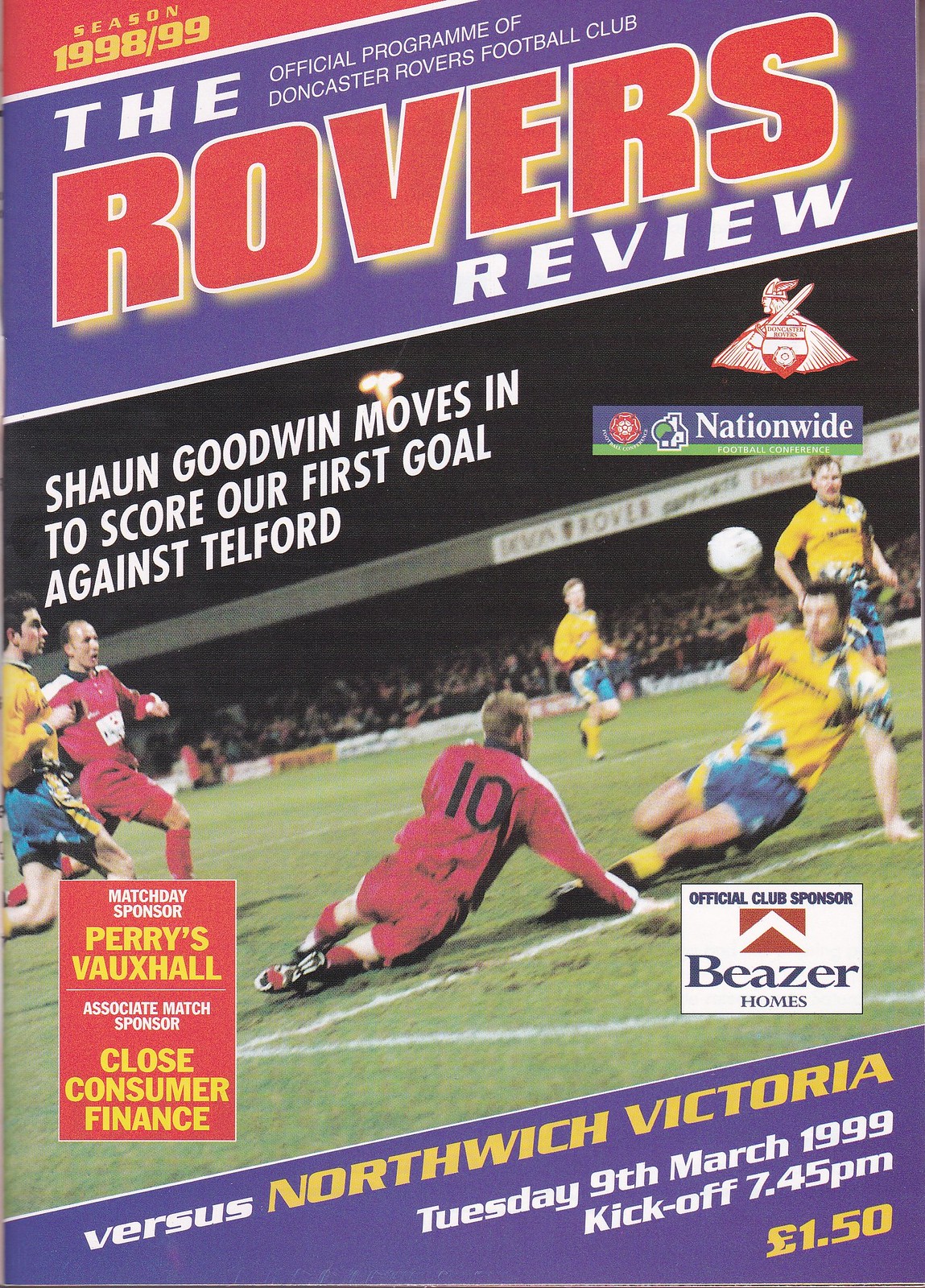The image appears to be a detailed cover of a magazine or program for the Doncaster Rovers Football Club's 1998-1999 season. The title "The Rovers Review" is prominently displayed in bold, red font with gold shadows, accompanied by the subtitle "Official Program of Doncaster Rovers Football Club" in white. The cover features vibrant colors, including green, red, purple, yellow, and white.

At the top, starting in the left corner, there is a white line that forms a triangle cut off in the center. This segment reads "Season 1998-1999" in gold letters against a red background. Below it, a thick, purple rectangle spans the width, reinforcing the title. 

The main image shows a somewhat distorted action shot of men playing soccer on a field, with some players on the ground and others running. One team is in red and the other in yellow, with a crowd visible in the distance. Text over the photo reads, "Sean Goodwin moves in to score our first goal against Telford."

The bottom section lists details of the upcoming match: "Versus Northwich Victoria, Tuesday, March 9th, 1999, Kick-off 7.45 p.m." It mentions that the program is priced at £1.50 and notes the official club sponsor, Beezer Homes.